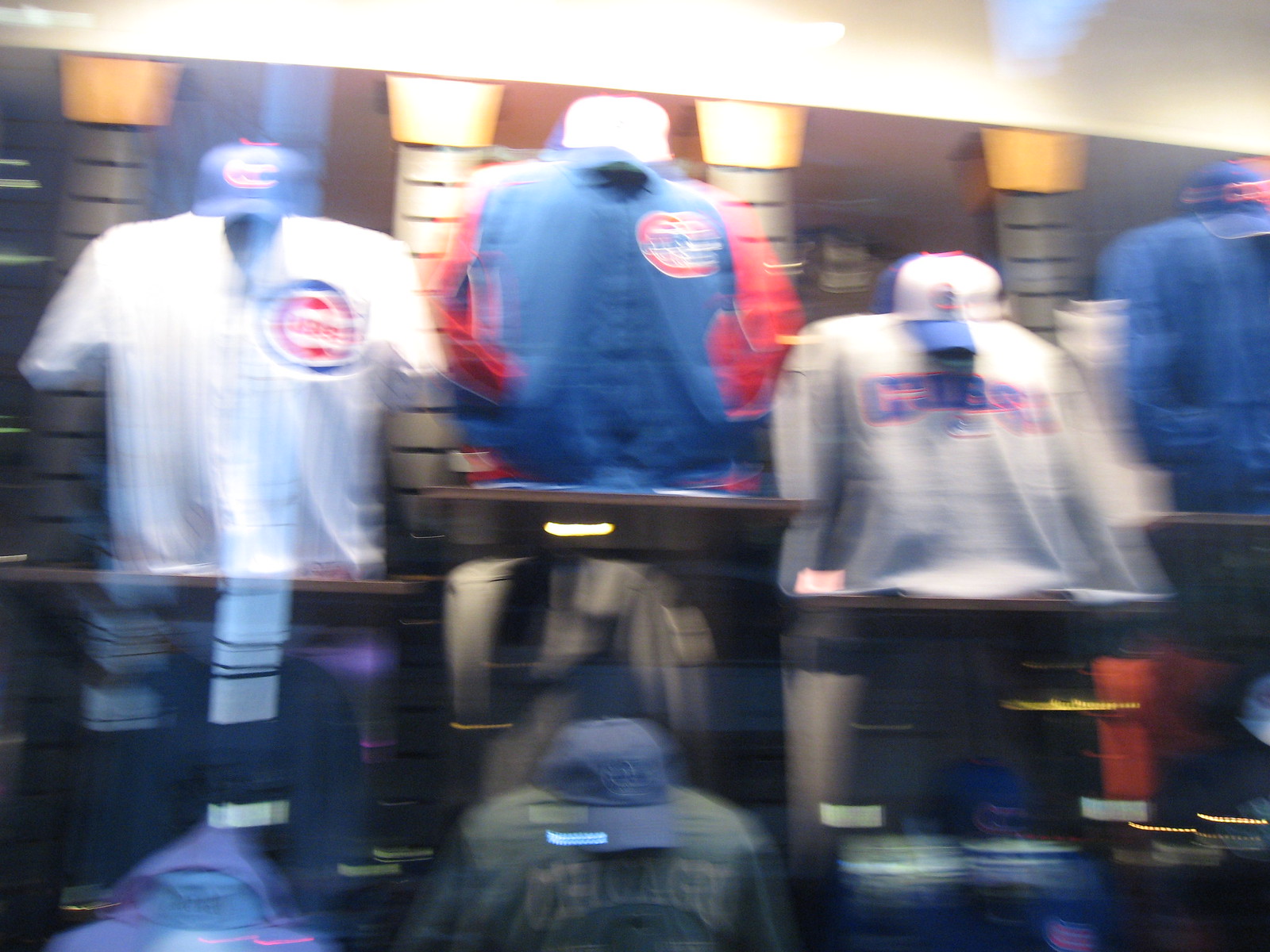The image appears to capture a distorted, blurry photograph of a clothing retail store, specifically selling Chicago Cubs merchandise. The distortion seems to be due to camera shake, possibly taken quickly with an older phone, resulting in poor detail and various light distortions. The upper two-thirds of the image prominently display several mannequin torsos wearing different Chicago Cubs gear: a white Cubs jersey with a blue hat, a blue Cubs jacket with red sleeves, a grey Cubs sweatshirt with a white hat, and another unidentifiable item with a blue Cubs hat on a blue stand. These mannequins are set against a brown wall illuminated by four lights. The lower part of the image vaguely shows more merchandise on shelves, including additional clothing items and hats, though their details are too indistinct due to the blurriness. Some reflections in the image suggest this photo could have been taken through a window. The store seems to have a black wall in the background with a white ceiling accented by lights and possible orange designs.